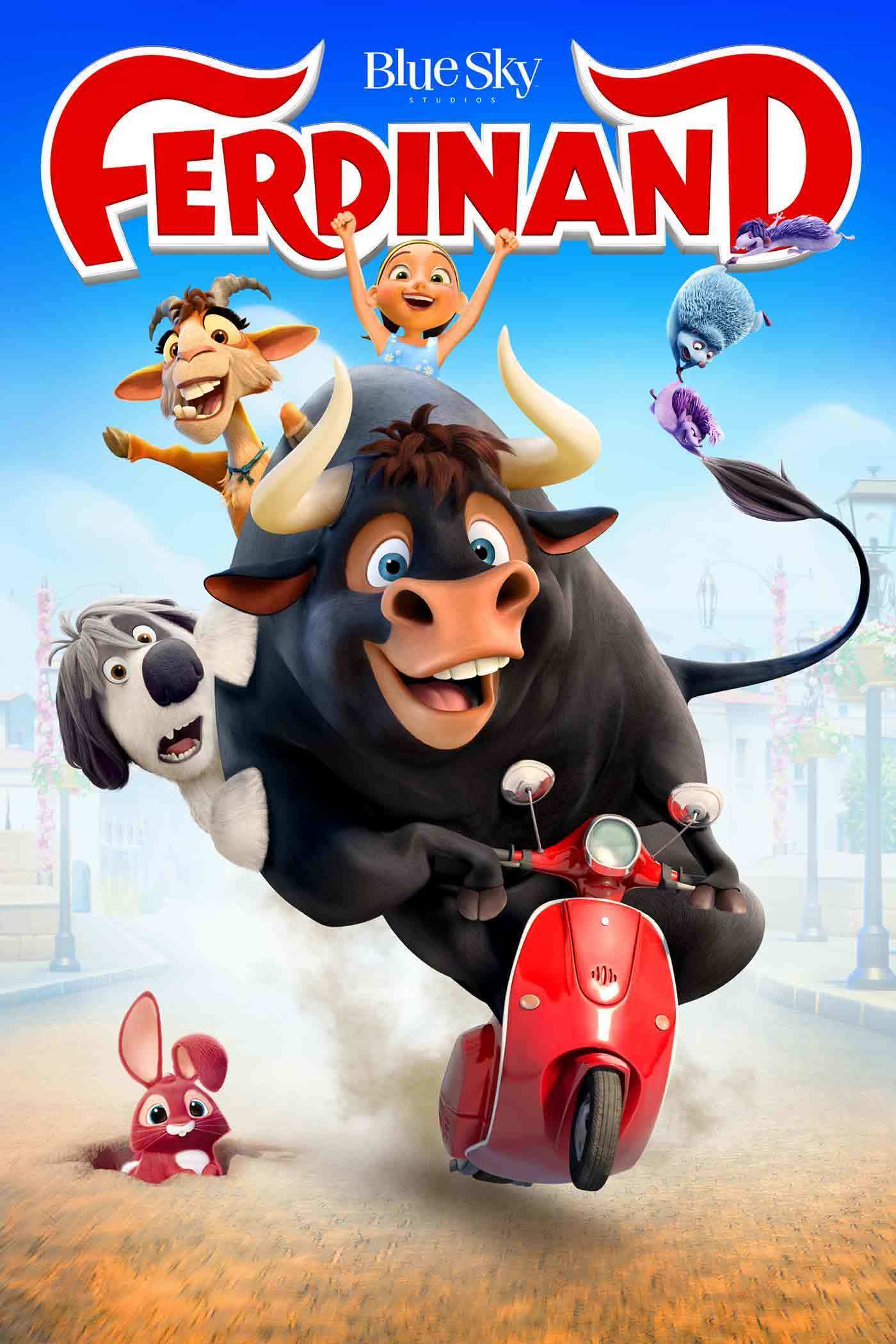The movie poster features a vibrant illustration against a blue background, with the words "Blue Sky" in white at the top, followed by "Ferdinand" in bold red letters. Below the text, a large, smiling black bull with blue eyes is prominently riding a red scooter. On his back, the bull carries an animated ensemble, including a young girl, a white dog, and a goat, all smiling. His tail juts out to the right and supports a light blue possum along with a couple of other purple furry animals. The bull’s jovial expression is complemented by his wide face and big nose. Beneath the scooter, the ground resembles a brown street, where a red bunny rabbit pops its head up from the bottom left of the image. The background showcases a faint sidewalk and several street lamps, subtly faded into the blue canvas, enhancing the dynamic and cheerful atmosphere of this captivating scene.